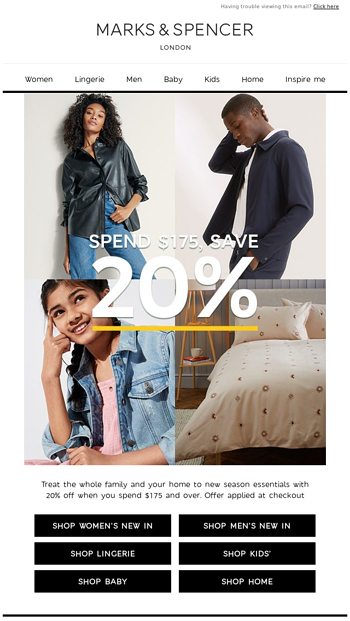Here is a cleaned-up and highly detailed descriptive caption for the image:

---

This portrait-style vertical screenshot captures the email template of the Marks & Spencer website. At the top, a white banner houses the iconic Marks & Spencer logo in black font, accompanied by a notification that reads: "Having trouble viewing this email? Click here." This indicates the website's layout is designed for email correspondence. 

Directly below the banner, several category links are prominently displayed, including Women, Lingerie, Men, Baby, Kids, Home, and Inspire Me. The central section of the template features a four-panel photograph highlighting various Marks & Spencer products. The first panel showcases a woman in a stylish leather jacket, the second panel shows a man dressed in a sleek suit blazer, and the third panel presents a young teenager wearing a trendy jean jacket. The fourth panel diverges from apparel and displays a white bedspread adorned with black moon and sun designs.

Beneath the image collage, a promotional text reads: "Treat the whole family and your home to new season essentials with 20% off when you spend $175 or over. Offer applied at checkout." This is followed by a series of black buttons with white text, each linking to different sections of the shop: Shop Women's New In, Shop Men's New In, Shop Lingerie, Shop Kids, Shop Baby, and Shop Home.

---